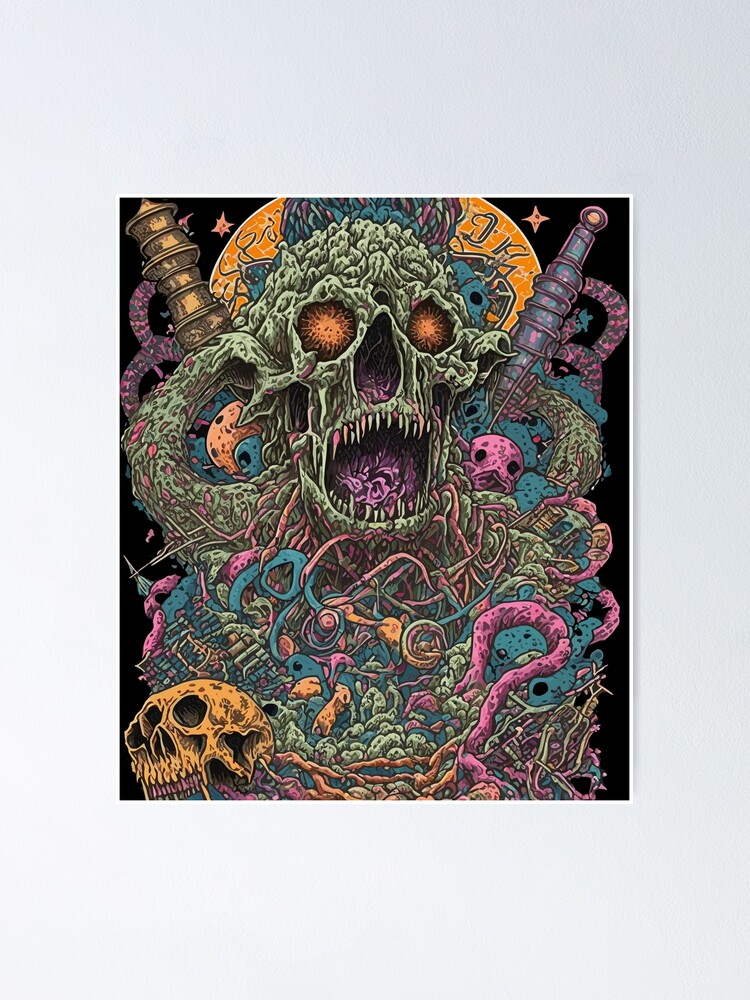The image is a vibrant and detailed poster depicting a psychedelic painting of a ghastly green skull embellished with sharp, fang-like teeth. The skull’s eye sockets are filled with bright yellow-orange explosions, resembling firecrackers. Two swords cross behind the skull, enhancing the menacing aura. Green snakes coil around the skull’s shoulders, merging seamlessly with its hue. The nose and jaw areas of the skull appear hollow, further adding to its eerie demeanor. Surrounding the main skull are smaller, vividly colored skulls, including a purple one near its mouth and an orange one in the bottom left corner. The background is a chaotic blend of colors and imagery, featuring other skeletal faces, possible creatures, and worms emerging from the scene. The overall palette includes pink, brown, yellow, orange, purple, golden, black, and white, creating a strikingly colorful and intricate composition. The artwork is full of unsettling details, with the mouth open wide and seemingly filled with worms, adding to its grotesque impact. This piece demonstrates an incredible level of detail and craftsmanship, making it both intriguing and nightmarish.